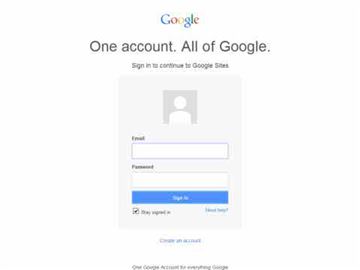The image is a small, shrunken down screenshot of a Google sign-in page, not to scale and barely legible even on a small smartphone. At the top, there is a prominently displayed Google logo followed by the text "One account. All of Google." The page prompts users to sign in to continue to Google sites. Below this header is a grey square featuring a simplistic white icon of a person—essentially a dot representing the head and shoulders.

The first input field is designated for entering an email address, followed by a second field for the password. The "Sign In" button is visible beneath these input fields. Despite the overall blurriness, there's a checkbox below the "Sign In" button, which is currently checked, accompanied by the text "Stay logged in."

To the right of the checkbox is some blue text, but it's unreadable due to its small, pixelated size. Further down the page, some more text appears, potentially indicating options like "Close my account" or similar, although this too is difficult to decipher given the extreme blurriness and small font size. The bottom of the page reiterates the message: "One Google account for everything Google," although reading this text is challenging due to its pixelated nature. The background of the page is white, but the entire image is highly blurry and considerably shrunken, making the sign-in area difficult to read.